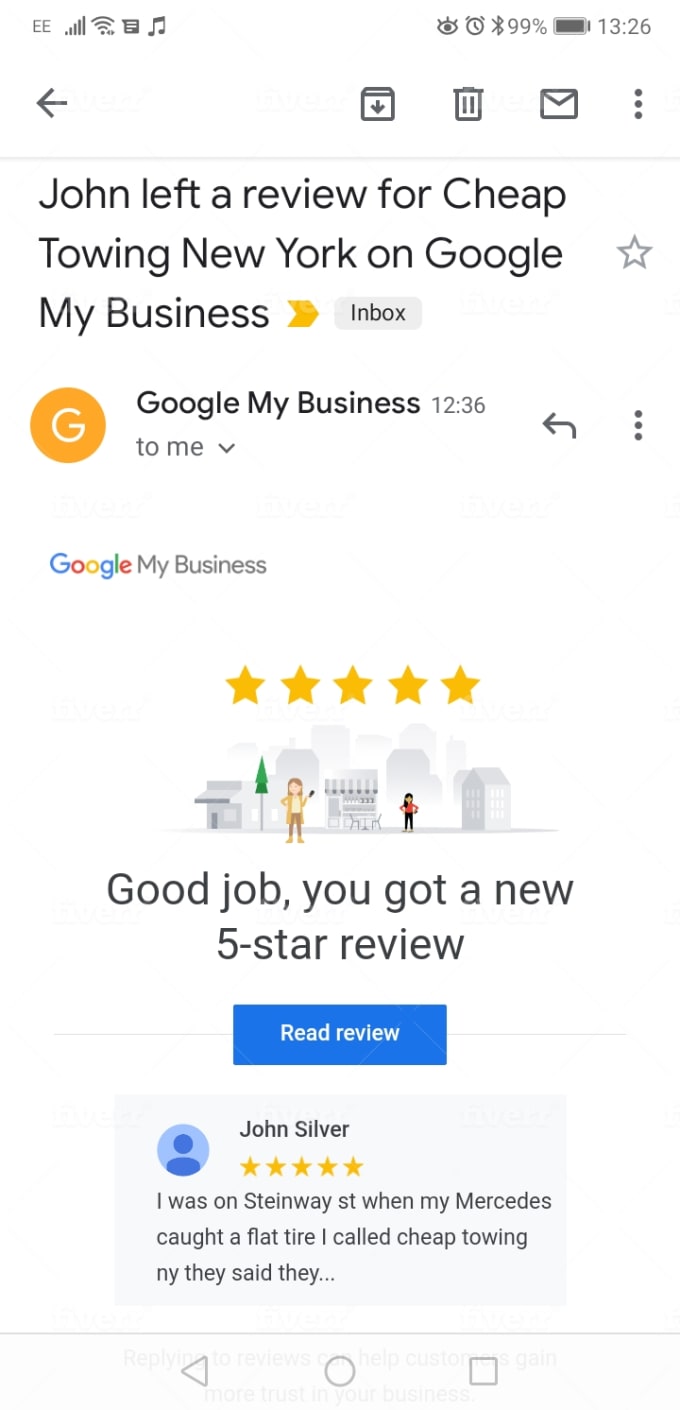A detailed caption for the image would be:

A screenshot of a cell phone displaying an email with a notification for a business review received through Google My Business. At the very top left corner, common cell phone icons can be seen, including the wireless signal and cellular connection indicators. On the top right, there is a Bluetooth logo next to "99%" indicating battery life, followed by a battery icon. 

The email's subject line reads, “John left a review for Cheap Towing New York on Google My Business," with the word "Inbox" highlighted, indicating the current mailbox being viewed. Just below the subject line, a yellow circle with a white letter "G" inside identifies the sender as Google My Business. The email timestamp is marked as “12:36.” The recipient is labeled as "To: Me" with an adjacent drop-down arrow that likely expands additional recipient details. 

Below, prominently featured, is the Google logo next to "My Business", followed by a noteworthy five-star rating, each star filled with yellow. Accompanying this is an image of a city street backdrop, complete with buildings and two individuals standing in the foreground and background, both facing forward. 

A congratulatory message in large text states, "Good job, you got a new five-star review." Beneath this is a blue button with white text that says "Read Review." Following the button, the review is displayed in a rectangular box. The upper section of the box features a circular icon representing a person, labeled "John Silver," along with another five-star rating, each star filled in yellow. The review text begins, "I was on Steinway Street when my Mercedes caught a flat tire. I called Cheap Towing NY. They said they..." and trails off with an ellipsis indicating more text is available upon expanding the review.